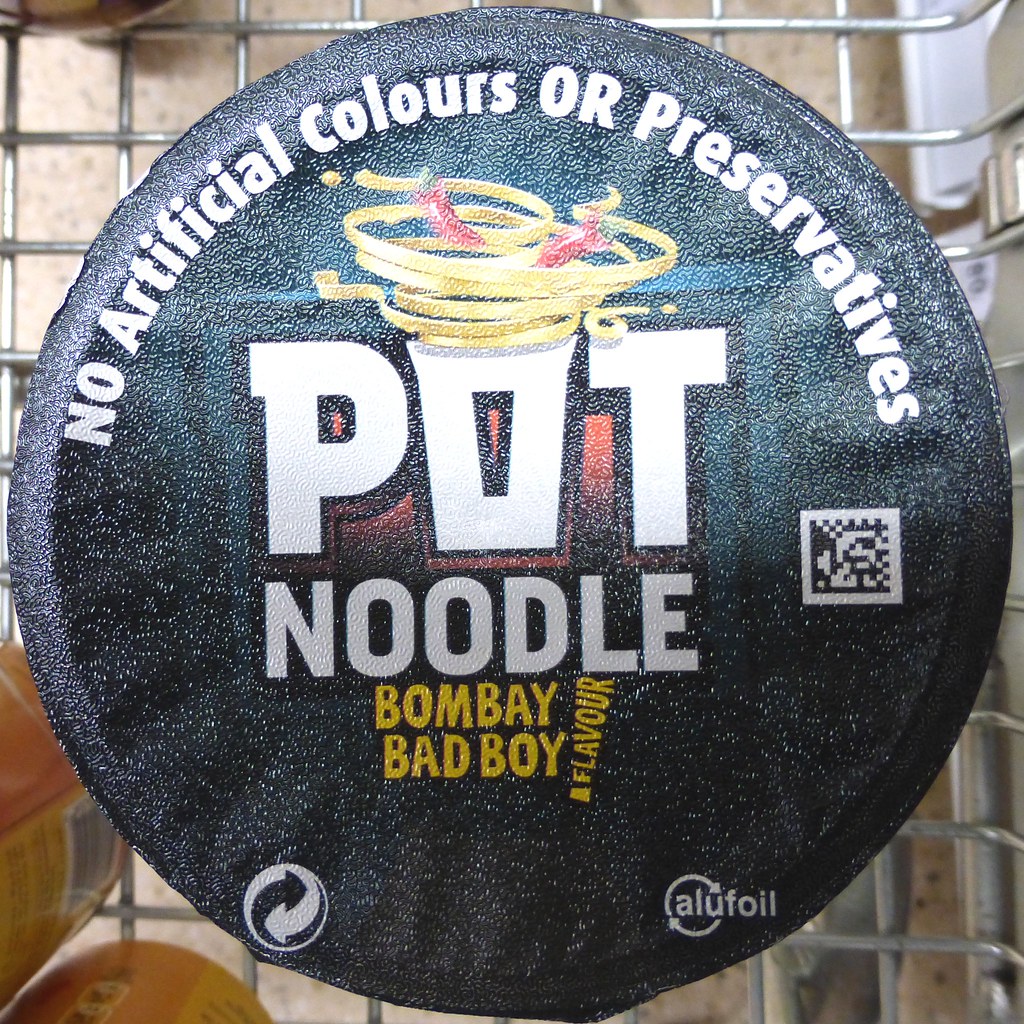The image shows a top view of a Pot Noodle container, specifically the "Bombay Bad Boy" flavor. The container has a round, black, and metallic-like foil lid that is shiny. Prominently displayed at the center, in white text, is "Pot Noodle," with swirling noodles and red peppers above the letter 'O'. Just below the main label, the flavor "Bombay Bad Boy" is written in yellow, alongside a QR code. Encircling the top edge of the lid, it reads "no artificial colors or preservatives" in white text. Towards the bottom, on the left, two recycling arrows—one black and one white—are seen nestled together, and on the right, the label "alu foil" is present indicating the use of aluminum foil. The container is positioned within a grocery cart, evidenced by the metal grid of the cart visible beneath it, along with glimpses of the store's floor. Additionally, there are other items nearby, including orange-colored containers. The image captures an overhead perspective, making the lid appear as though it's standing upright.